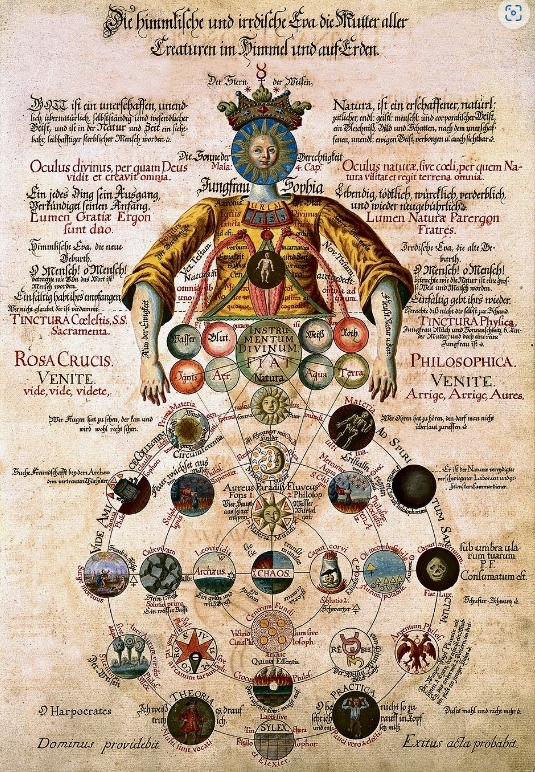This detailed medieval-looking poster, presented on an aged parchment background, resembles a page from a vintage book. It features ornate writing in black and red, both in cursive and non-cursive, and is titled in a distinctive medieval font. Central to the image is a crowned figure with a golden sun for a head, set against a blue backdrop, symbolizing royalty. The crown, adorned with three golden spikes, sits atop this radiant head. The figure's neck and skin are outlined in a bluish-gray hue, complementing its yellow long-sleeve shirt or dress. 

This figure extends its arms outward, and its torso is composed of numerous circles. Each circle contains various intricate images, shapes, or symbols, including depictions of trees, dragons, DNA strands, and a sun. The arrangement of these circles gives the impression of the figure's body and dress, forming a cohesive round shape that contributes to its queenly appearance. Notably, one central circle labeled "Chaos" appears below the head, close to another labeled "Fiat," denoting a sense of cosmic order and disorder. 

The detailed diagrams and text are adorned with multiple ornate letters, and the whole graphic is flanked by extensive writings on either side in what appears to be Latin or German, adding to its mysterious and scholarly aesthetic. The phrase "Dominus Pervit" is inscribed at the bottom, further enhancing the poster's vintage and authoritative allure.